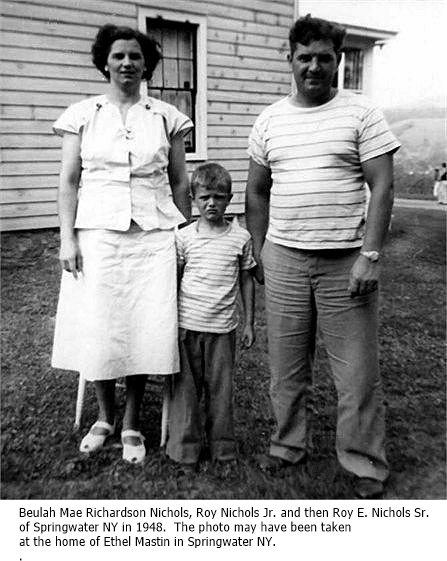This black-and-white photograph from 1948 captures the Nichols family of Springwater, New York, possibly taken at Ethel Masten's home. Featured in the image, from left to right, are Beulah Mae Richardson Nichols, a young woman dressed in white, and Roy E. Nichols Sr., a clean-shaven man clad in jeans and a striped short-sleeved shirt. Centered between them is their son, Roy Nichols Jr., around seven or eight years old, wearing a striped shirt and jeans. They are standing outside on the grass, likely in a front yard, with a house and part of a car visible in the background. Beulah may be seated, suggested by the legs of a chair behind her. None of the family members are smiling, with the boy notably frowning. The image is marked with the names and details of the family members at the bottom.